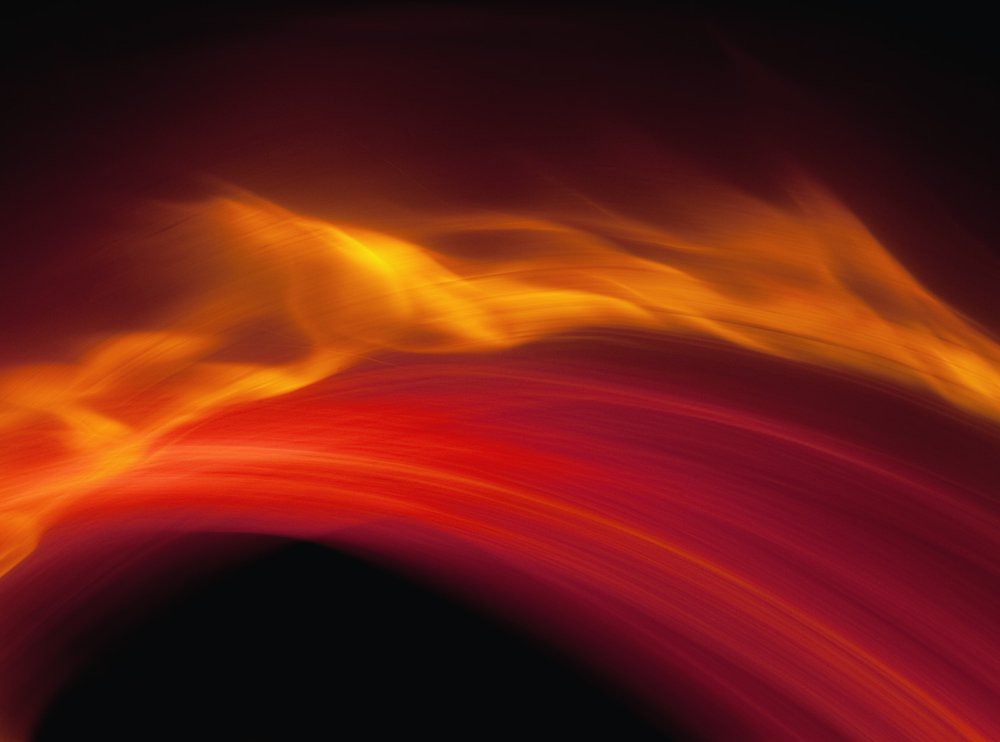The image depicts a dramatic scene with a black background, featuring an intense display of fire in a half-circle or arc shape. This fiery arc extends across the middle and lower parts of the image, reaching from the bottom left toward the bottom right. The base of the fire comprises solid, dark red bands, resembling tires or a structured form. Above these bands, wild flames in shades of orange and yellow seem to dance and stream upwards, creating a vivid contrast against the dark backdrop. The fire appears as if it's racing or being blown by some force, adding a dynamic sense of movement to the scene. The entire composition combines shades of black, maroon, and fiery reds and oranges, evoking the image of a fiery landscape or even the surface of a blazing sun.